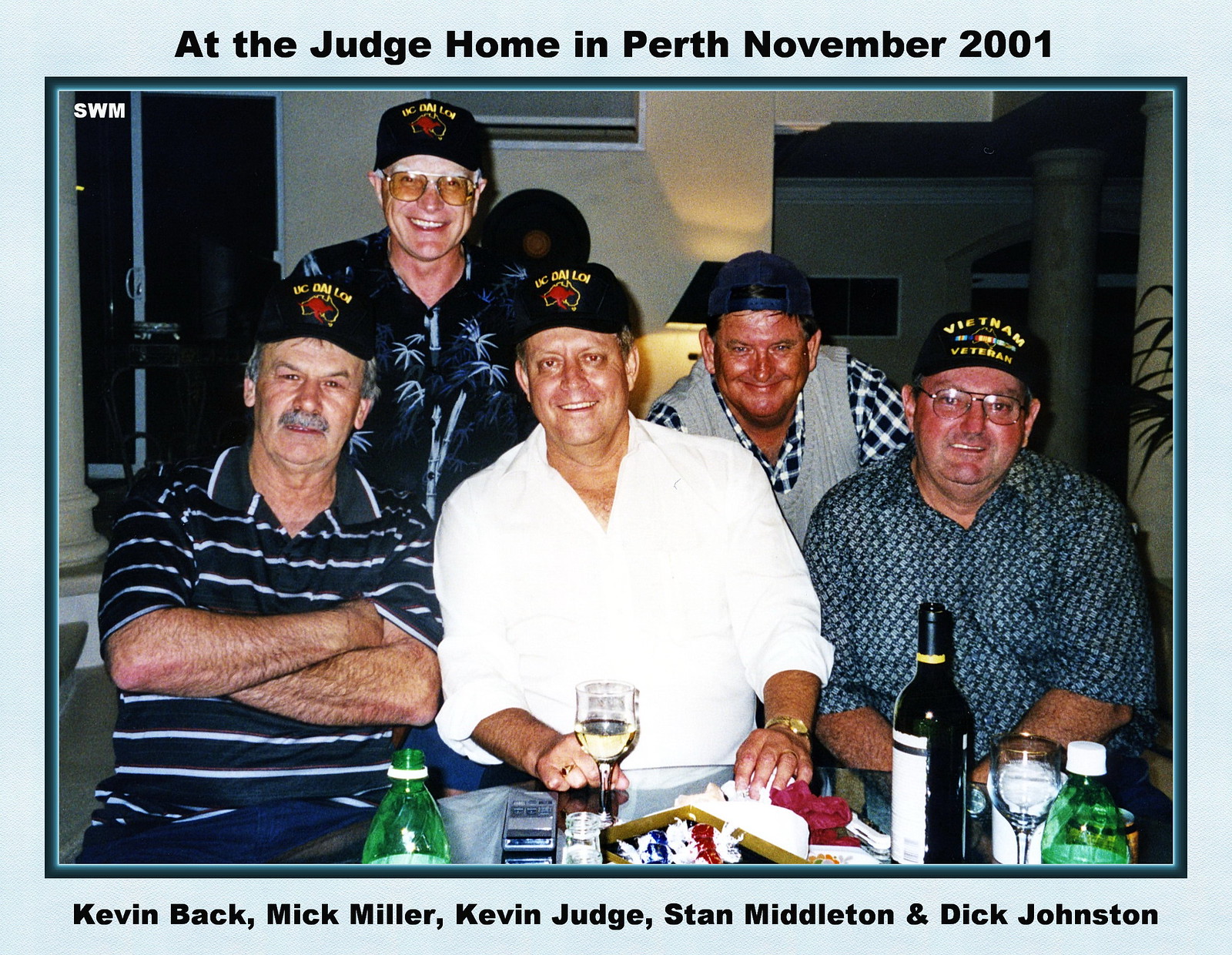This vibrant, full-color photograph captures a joyous indoor veterans reunion held at the Judge Home in Perth, November 2001. Enclosed within a light blue border and a darker blue inner trim, the image’s top border bears the caption in black print, while the bottom border lists the names of the men from left to right: Kevin Back, Mick Miller, Kevin Judge (the host), Stan Middleton, and Dick Johnson.

Seated around a table adorned with liquor bottles, wine glasses, cigarettes, and gambling utensils, the five older gentlemen are clad in diverse attire but united in camaraderie through their Vietnam veteran hats. Kevin Back, on the far left, appears around 50 years old, with gray facial hair and crossed arms, wearing a black shirt with white stripes and blue pants. To his right stands Mick Miller, donned in a black Hawaiian shirt with white and gray palm trees, glasses, and a red hat featuring a kangaroo logo.

Hosting the gathering, Kevin Judge sits at the center, grinning with short gray hair, a white shirt, a watch on his left wrist, and a ring on his right hand, next to a glass of wine. Behind Kevin Judge to the left, Stan Middleton sports a blue hat turned backward, a gray vest, and a white and blue pleated shirt. At the far right, Dick Johnson, wearing glasses and a blue "Vietnam Veteran" hat with a small map of Australia, smiles while donning a gray patterned shirt.

All are captured smiling broadly, embodying the spirit of reunion and shared history, with their “UC Dai Loi” hats, symbolizing their connection, and topped off with specified banners detailing their names and the event's location.